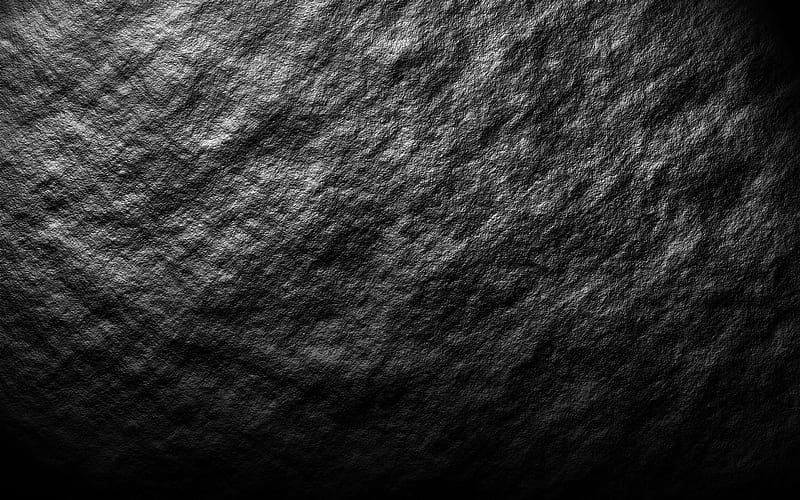This photograph captures a close-up view of a smooth, rocky surface, likely part of a cave wall or stone face. Dominated by uniform gray tones, the image reveals the stone's weathered yet smooth texture, with subtle recesses and outcroppings creating an uneven, bumpy appearance. The primary light source, coming from the upper left, casts shadows that darken the bottom and upper right portions of the image, forming a circular pattern of illumination across the stone. The minimalist aesthetic and lack of additional features or colors emphasize the natural, earthy character of the stone, with no text or other elements to distract from its texture and form.